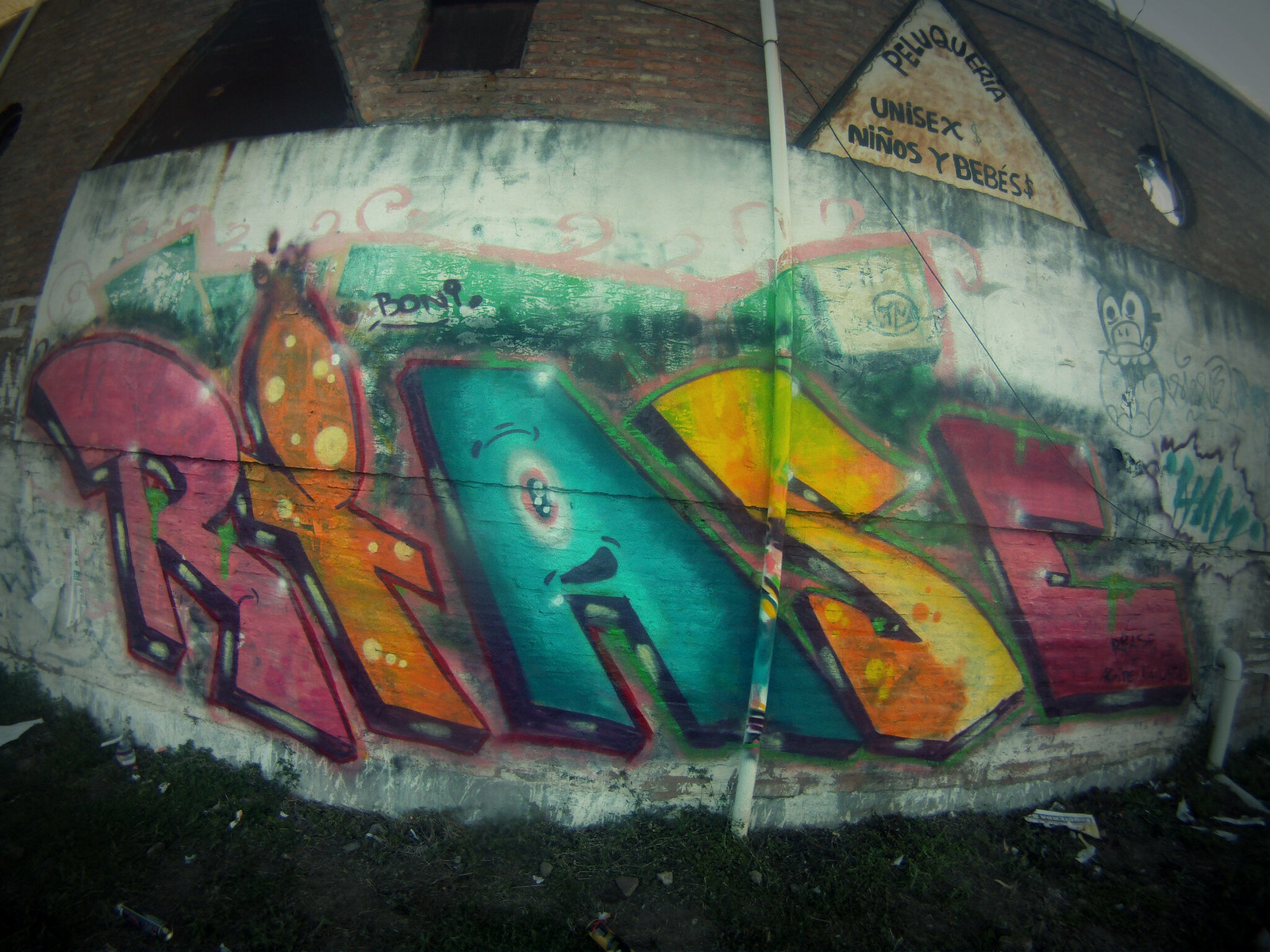A dynamic pop art painting features vibrant, colorful lettering against a light background. The artwork is bordered with a brownish-black trim at the top and a black base. Dominating the canvas are four large, eye-catching letters; a pinkish "R" on the left, an orange "T" with a dot above it, a teal "A," and a yellow "S," followed by a pink "E." Intricately scribbled graffiti weaves behind the letters, adding texture and depth. At the top, amidst the brown trim, a sign prominently displays the text "Pell Quill Area, Unisex, Minos, Ibibisa." Despite the hint of structured typography, no specific signage is present within the scene itself.